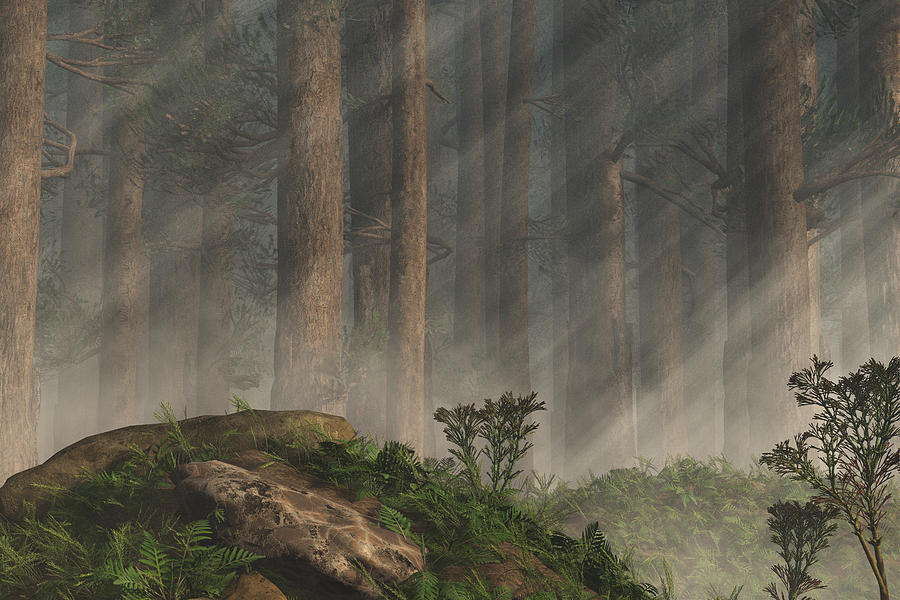This detailed piece of artwork, a painting or possibly digital art, depicts a serene, mystical forest. The scene is softly illuminated by beams of sunlight filtering diagonally throughout the frame, casting a hazy glow on the wide-trunked, tall trees that dominate the background. These trees, possibly pines, have bare, thick trunks for the most part, with occasional branches devoid of leaves, and their tops extending out of the frame. In the lower left corner, a rock formation is lush with various green plants and ferns. A mossy hill filled with jutting rocks and more ferns adds texture and depth to the composition. In the lower right-hand corner, two small bushes emerge from the ground, and a little flower bush grows atop one of the boulders, though color is largely subdued across the scene. The interplay of gray and white sunlight beams intertwined with the tranquil tones of browns and greens enhances the dreamlike quality of this fantastical forest, devoid of creatures or people.